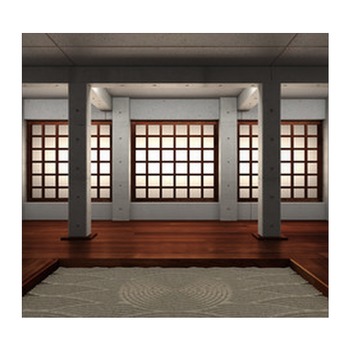This is a detailed photograph, possibly a computer-generated image, of what appears to be a Japanese-style room within a larger, sophisticated building. The room features a striking hardwood floor, rendered in warm, varying shades of brown and tan. In the center of the floor, there's a significant, slightly sunken mat area with a lighter shade, creating a subtle contrast that might suggest a specialized purpose, like a dojo or another traditional setting.

Symmetry and balance define the room's design. The far wall is adorned with three large square windows, each framed intricately with wooden borders and divided into smaller symmetric panes. These windows allow light to flood the room, though the external view is obscured. Supporting the low ceiling are two robust vertical columns situated centrally, complemented by matching pillars against the wall, emphasizing structural integrity.

The color palette captures an array of natural tones—whites, off-whites, blacks, grays, and multiple earthy browns—giving the room an inviting but refined atmosphere. The careful composition and centered perspective of the image highlight the room's harmonious and well-balanced architectural elements, suggesting both functionality and aesthetic appeal.